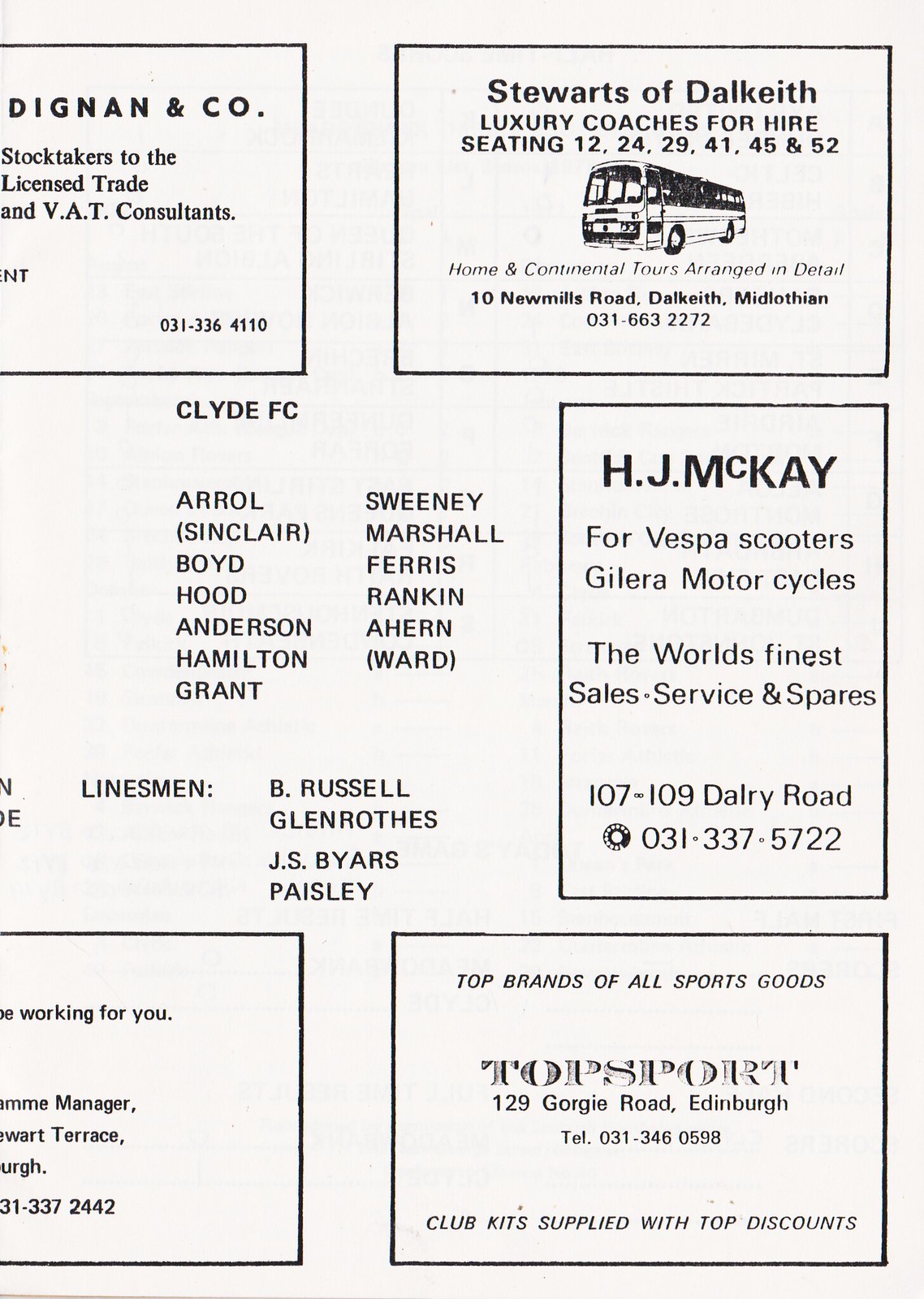The image is a scanned page from a vintage magazine or newspaper, positioned as the right half of a larger spread, with parts of adjacent boxes visible. Dominating the center is a list of soccer player names from Clyde FC, including Errol, Sinclair, Boyd, Hood, Anderson, Hamilton, Grant, Sweeney, Marshall, Ferris, Rankin, Ahearn, and Ward, along with linesmen B. Russell, Glenn Rothers, and J.S. Byers from Paisley. Surrounding this central column are several black-and-white advertisements, each enclosed in simple rectangular borders. At the top right, we have Stewart's of Dalkeith, which offers luxury coaches for hire with seating capacities ranging from 12 to 52, including details for tours and contact information. Midway down the right side is an ad for H.J. McKay, promoting Vespa scooters and Galera motorcycles, highlighting their sales, service, and spares. Another visible ad is for Top Sports, offering top brands of sports goods with an address in Edinburgh. The stark, monochromatic design features black text on a white background, enhancing the vintage feel of the page.